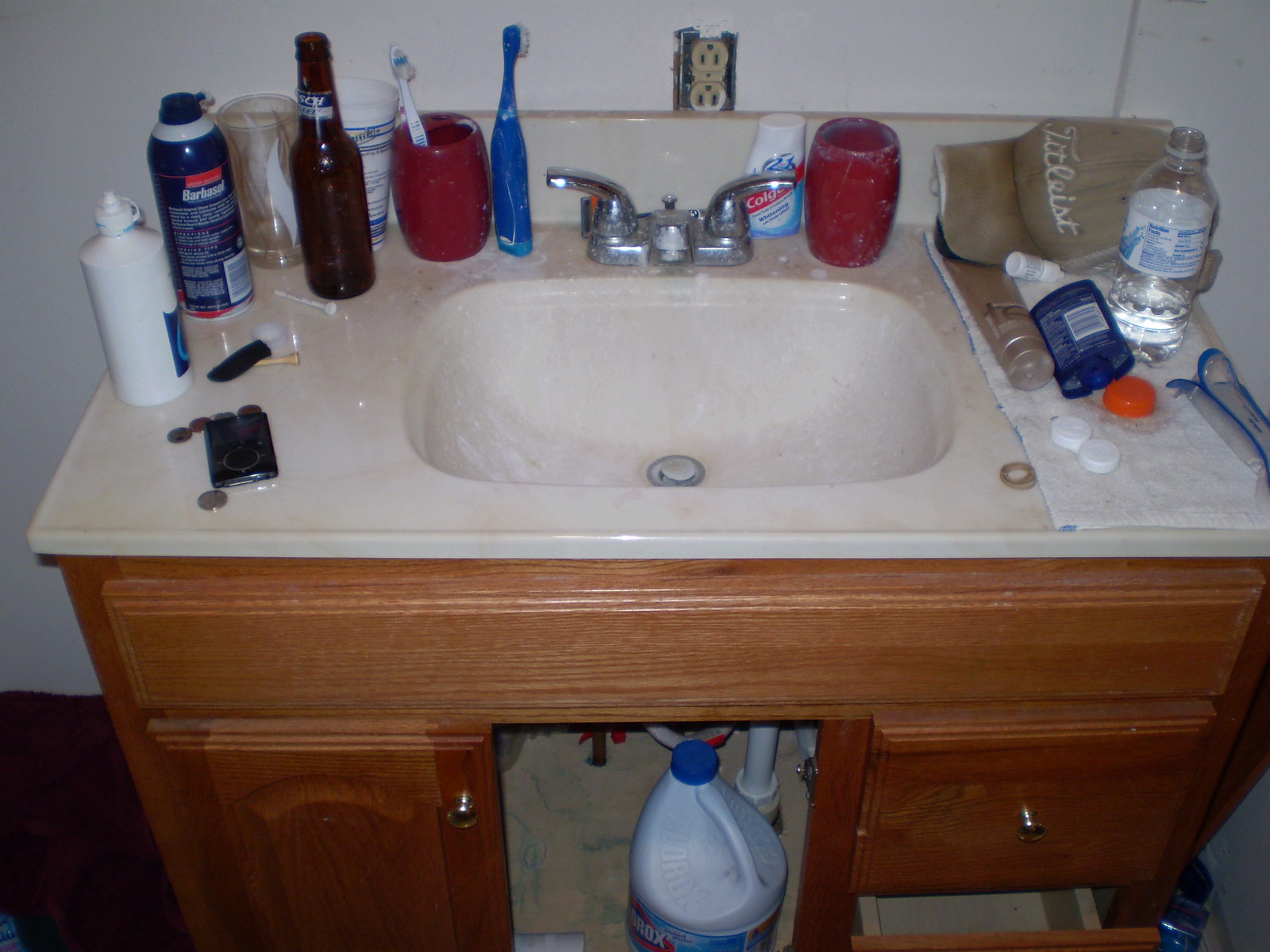The image is a color snapshot photograph taken in a bathroom, focusing on a sink set on a wooden base. The wooden base has both cabinets and drawers, with noticeable openings. Directly under the sink, nestled among exposed pipes, sits a bottle of bleach.

The countertop, an off-white marble hue, shows signs of wear and tear. A variety of bathroom items clutter the counter's surface: a wallet with loose change, a bottle of contact lens solution, a can of shaving cream, an empty beer bottle, a glass container filled with toothpicks, and a toothbrush cup with a toothbrush sticking out of it. An electric toothbrush stands next to the cup. Additionally, there are two tubes of toothpaste, a hat, a glass of water, and a stick of deodorant.

The sink itself is grimy, with visible white residue likely from shaving cream coating its interior. An open electrical socket is situated on the white background wall behind the sink, further emphasizing the disorderly state of the men's bathroom.